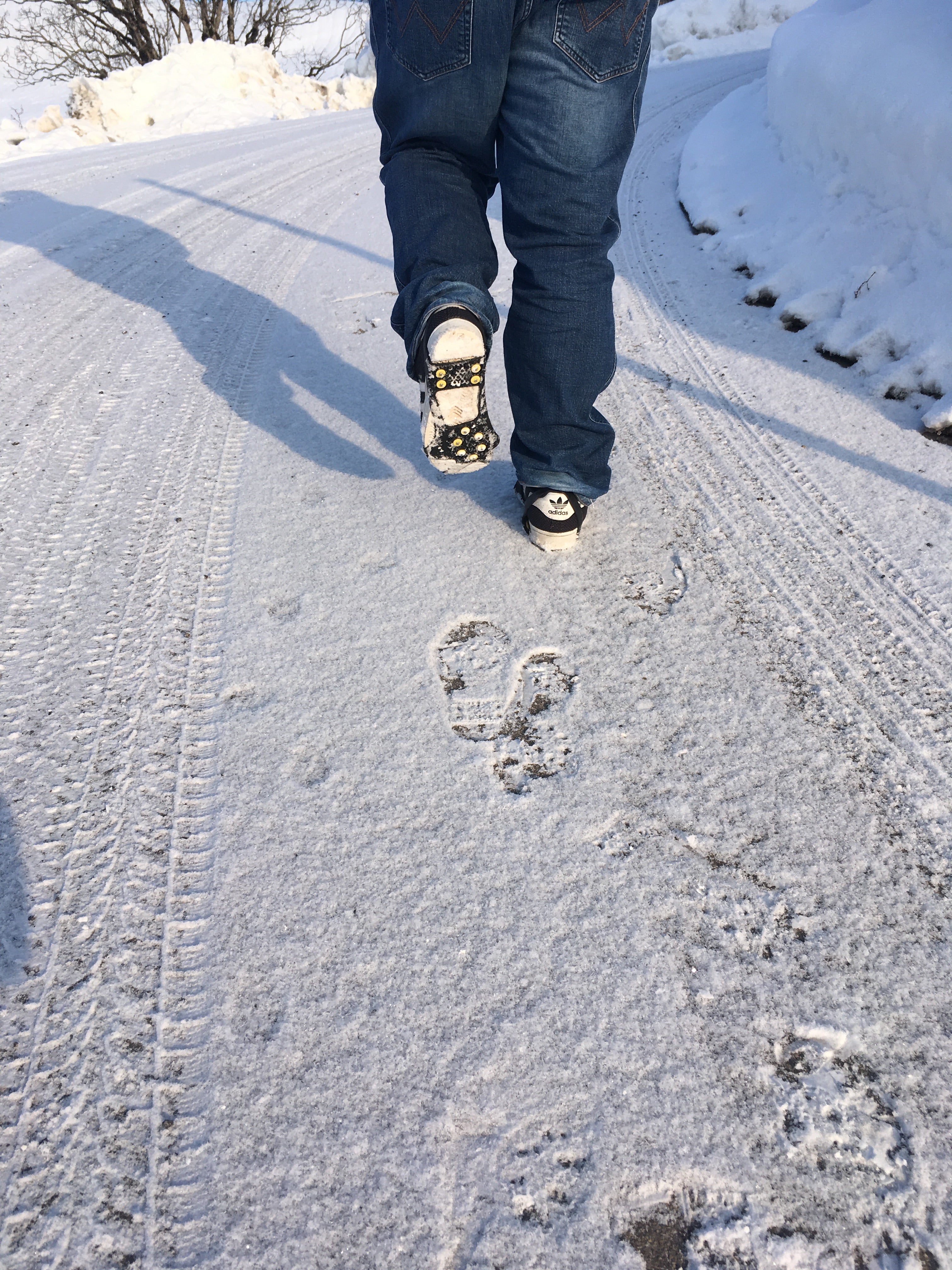In the photograph, we see a man walking away from the camera on a snow-covered road. Only the lower half of his body is visible, clad in blue denim jeans and white-and-black Adidas sneakers with yellow soles. The scene evokes a winter setting, highlighted by leafless trees in the background and a thick blanket of snow covering the ground. 

The road he walks on reveals partially-plowed snow, leaving tire tracks and various footprints, including animal tracks, to accompany the man's solitary path. His footsteps create a continuous trail in the fresh layer of snow, with his shadow stretching ahead of him, hinting that the sun is positioned behind his back. The road curves to the right about 20 to 30 yards ahead, leading the viewer's eye further into the serene, cold landscape.